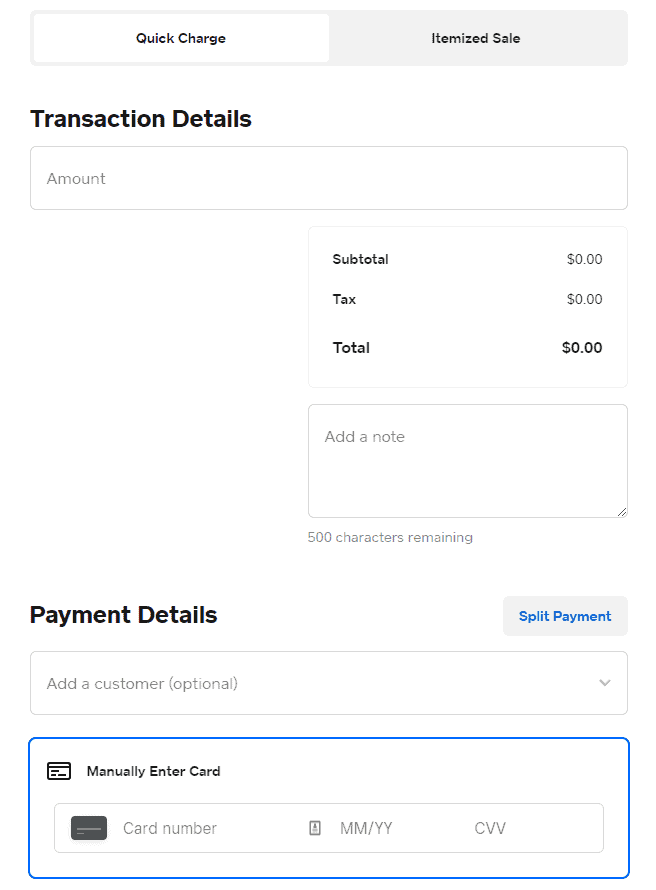This image, captured on a cellphone screen, showcases a transaction interface with various detailed sections. At the top, the screen is labeled "Quick Charge" in white, adjacent to "Itemized Sale" in gray, both housed within adjacent rectangles. Below this, the screen displays "Transaction Details," accompanied by a long, thin rectangle labeled "Amount," which is currently empty.

The middle section of the screen lists three key financial columns—"Subtotal," "Tax," and "Total"—each indicating an amount of $0.00. Near the bottom of this area, there is an option to "Add a Note," with a reminder that up to 500 characters can be used, though no note is currently present.

At the very bottom left, the interface highlights "Payment Details" in black. On the far right of this row, there's a clickable button labeled "Split Payment." Further down, another lengthy, slender rectangle invites the user to "Add a Customer," noted as optional. Finally, the screen offers a section to "Manually Enter Card" details, including "Card Number," "MM/YY," and "CVV."